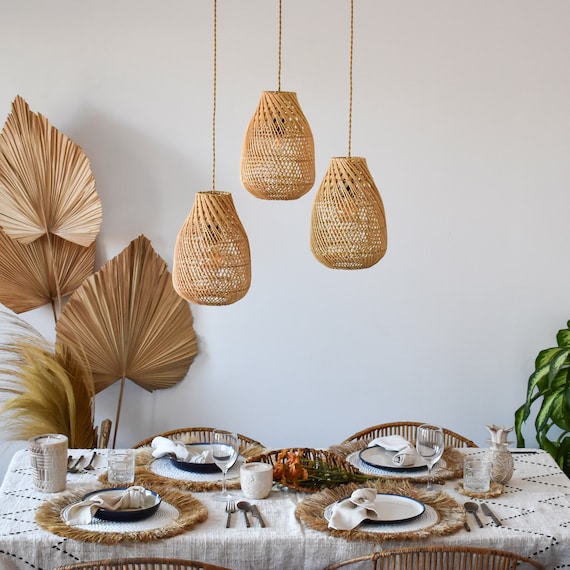This image showcases a beautifully arranged dining table set for a meal in a cozy, well-decorated space. The table, covered in a white linen tablecloth with navy blue embroidery, is surrounded by four wicker chairs with thin, curved backs featuring intricate woven patterns. Each of the four place settings includes a bamboo-style charger, a white plate, a multi-colored salad bowl, a white folded napkin, silverware, a wine glass, and a coffee cup. The centerpiece of the table is accentuated by a white and brown candle on one end and a decorative ceramic pineapple on the other. Overhead, three distinct chandelier lights hang, each encapsulated in a woven basket-like netting with a beaded string emerging from an open circle at the center. The backdrop features a taupe stone-colored wall adorned with large beige leaves and tall grass-like decorations, adding a natural, earthy feel to the setting. A lush green plant on the right side adds a pop of color and completes the inviting, elegant ambiance.